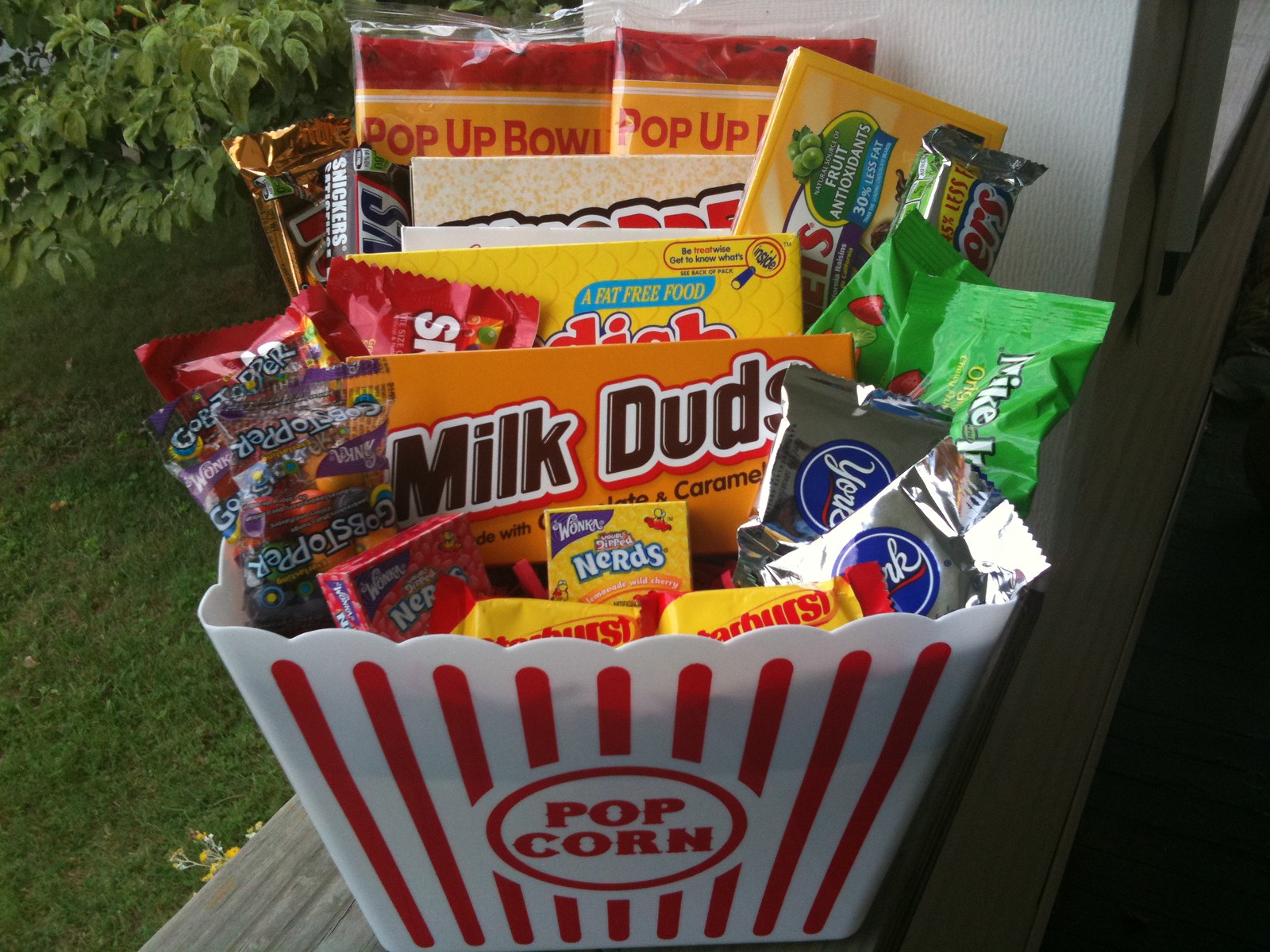This photograph captures a vibrant and eclectic display of candy inside a rectangular white plastic popcorn bucket with red vertical stripes. The bucket features a red-outlined circle at its center, emblazoned with the word "Popcorn" in classic red text, reminiscent of old movie theaters or county fairs. The bucket, situated centrally on a windowsill or some kind of outdoor ledge, is filled to the brim with a colorful assortment of treats. Among the visible candies are Mike and Ike's, Skittles, Whoppers, Milk Duds, Snickers, Twix, York Peppermint Patties, Starbursts, Nerds, Gobstoppers, Swedish Fish, and two packs of microwavable popcorn perched at the top. The candy packages add a kaleidoscope of colors to the composition, with vibrant reds, yellows, pinks, and greens making the display visually striking.

The setting appears to be semi-outdoors in the middle of the day, with a grassy area and a tree visible in the background on the left. The slight presence of greenery and the clear daylight give the scene a fresh, picnic-like atmosphere. The bucket sits on what could be a railing or park bench, enhancing the outdoor ambiance. The detailed candy display harmonizes with the simple, natural background, creating an inviting, nostalgic, and colorful image.